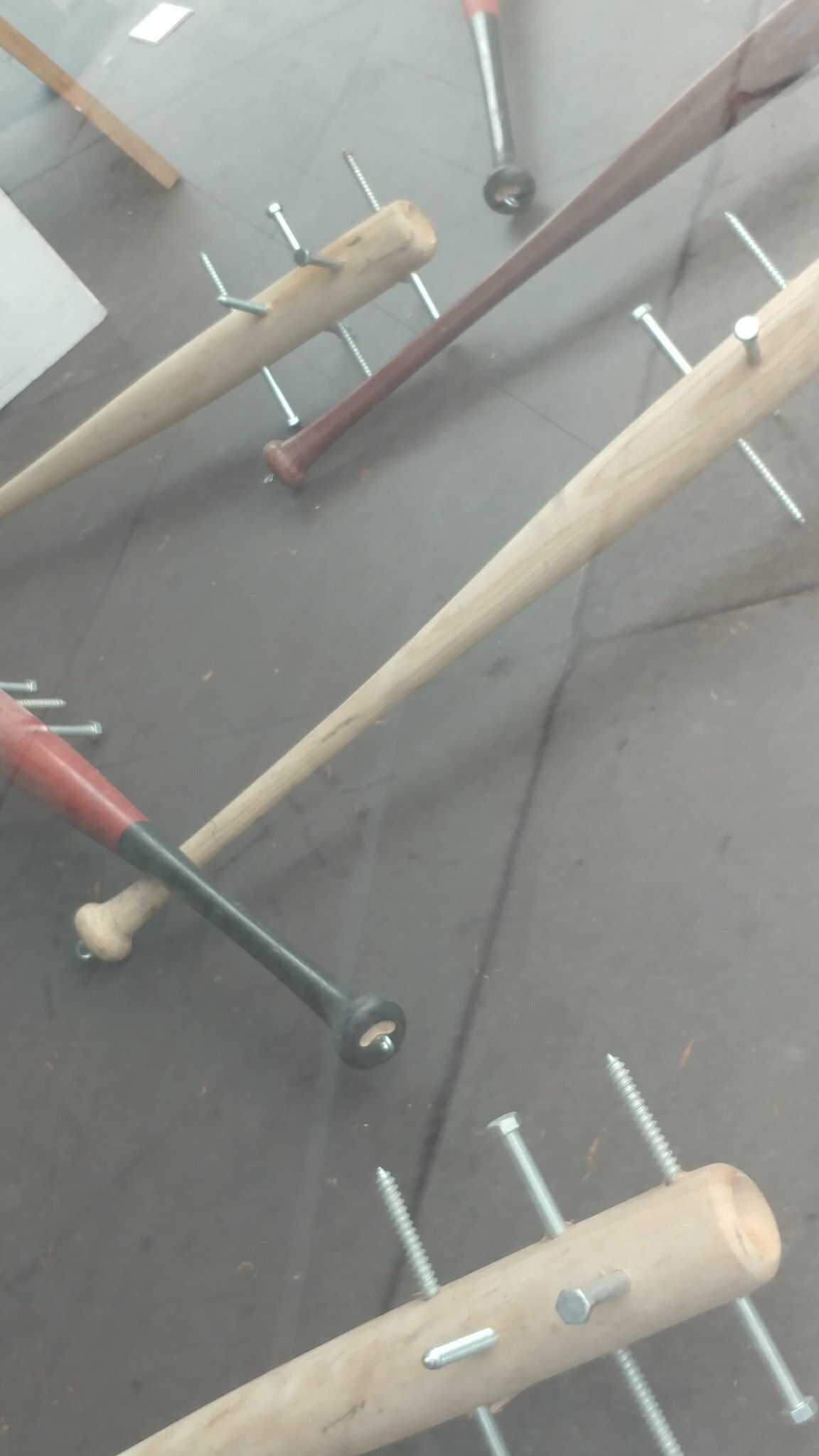This is a vertically rectangular color photograph depicting five baseball bats arranged on a large stone-tiled floor. Each bat has been turned into a formidable weapon by the addition of five 8-inch long screws drilled through them, with equal portions of each screw protruding on both sides of the bats. Three screws are inserted parallel to each other, while the remaining two are perpendicular to the first three, creating a grid-like pattern of metal points. The bats themselves vary in color: three are a light natural wood, one is a dark reddish-brown, and another has a striking black handle with a red body. The bats are positioned diagonally across the floor; four face to the right, while the red and black bat is oriented diagonally to the left. Amidst the arrangement, a loose screw is visible at the top edge of the photo, unconnected to any of the bats. The partial view of the bats emphasizes their menacing transformation into serious-looking weapons.